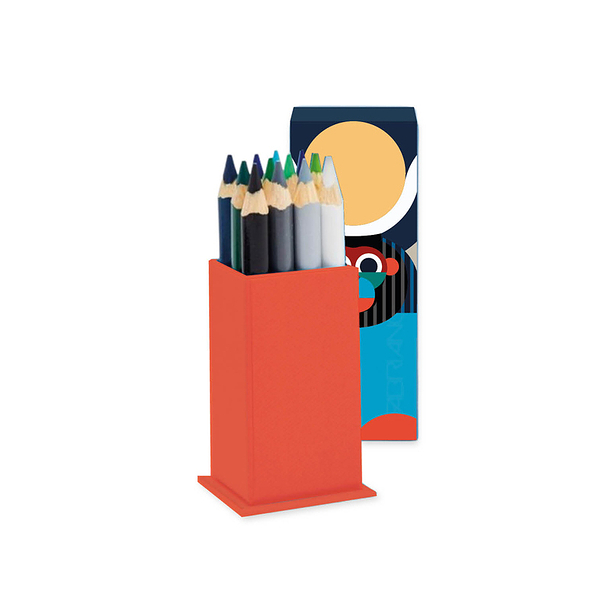The photograph features a long red box containing an array of sharp colored pencils organized upright. The pencils are in various colors including black, blue, green, dark gray, light gray, and white, with the solitary white pencil positioned in the right corner closest to the camera. Positioned behind the red box is a larger box that can slide over the red one to cover the pencils. This outer box showcases an abstract, minimalist illustration of an ape or monkey composed of simple blue, black, red, and white shapes. The creature's head is rounded and peanut-shaped, with basic circular eyes, and its body crafted from circles and ovals, giving it a cartoony feel. The entire scene is set against a stark, plain white background, with no additional elements in the frame other than the two boxes and the pencils meticulously arranged inside.